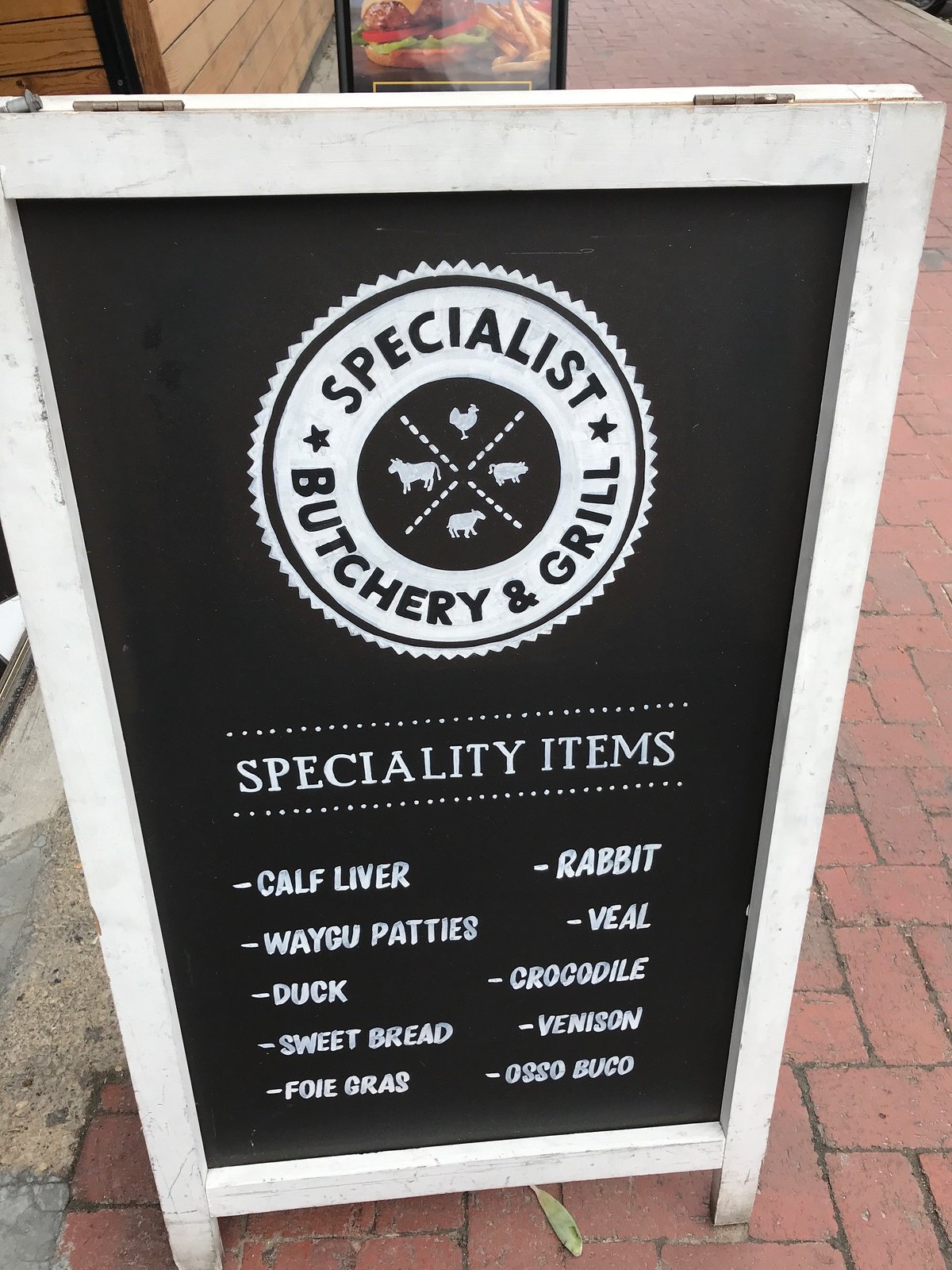The image portrays a sidewalk sign designed to catch the attention of passing customers for a business specializing in butchery and grill items. The A-frame sign is bordered in white wood and features hinges at the top for easy folding and storage. The display surface appears to be a high-quality print, giving it a sleek, professional look, although it mimics the style of a chalkboard.

At the top of the sign is a round logo with a dual-ring design. The outer ring is white, taking the form of alternating triangles, creating a gear-like effect. Inside the circle, depicted in white, are four animals: a cow on the left, a chicken at the top, a pig on the right, and a fourth animal that appears to be a sheep but could be mistaken for another animal. The name “Specialist Butchery and Grill” is emblazoned across the logo, separated by a star symbol, and an X made of dotted lines lies between the animals.

Below the logo, the sign advertises "SPECIALTY ITEMS" in bold, white capital letters. A dotted line borders this text both above and below, adding a distinctive touch. The items listed on the sign include an array of meats: on the left, “Calf Liver,” “Wagyu Patties,” “Duck,” “Sweetbread,” and “Foie Gras;” on the right, “Rabbit,” “Veal,” “Crocodile,” “Venison,” and “Ossobuco.” All text is presented in a manner that imitates chalk writing with remarkable clarity and precision.

The sign is situated on a brick walkway outside a business, hinting at a rustic or vintage establishment. In the background, there is another similar A-frame sign with an image of a burger and fries, showcasing the detailed layers of cheese, burger patty, tomato, lettuce, and bun, with fries on the side. This secondary sign continues the theme of mouth-watering food, evident from what can be discerned. Together, these signs create an inviting atmosphere that beckons potential customers to explore the culinary delights within.